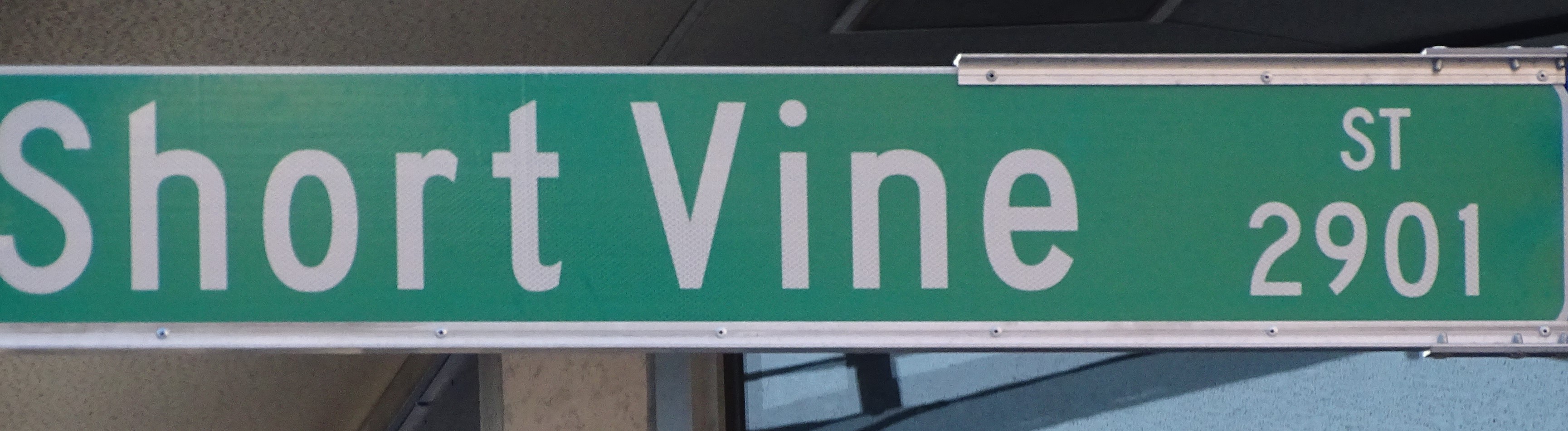"Close-up of a street sign that extends horizontally across the frame from left to right. The sign is green with a white border, featuring the text 'Short Vine' in white with a capital 'S' for 'Short' and a capital 'V' for 'Vine'. In the top right corner of the sign, there is an abbreviation 'ST' for street, and directly below this, the number '2901.' The right half of the sign is supported by a metal bar running along both the top and bottom, with visible small studs or screws securing it in place. The background is not clearly discernible, offering an ambiguous mix that could either be the underside of a bridge or the sky."